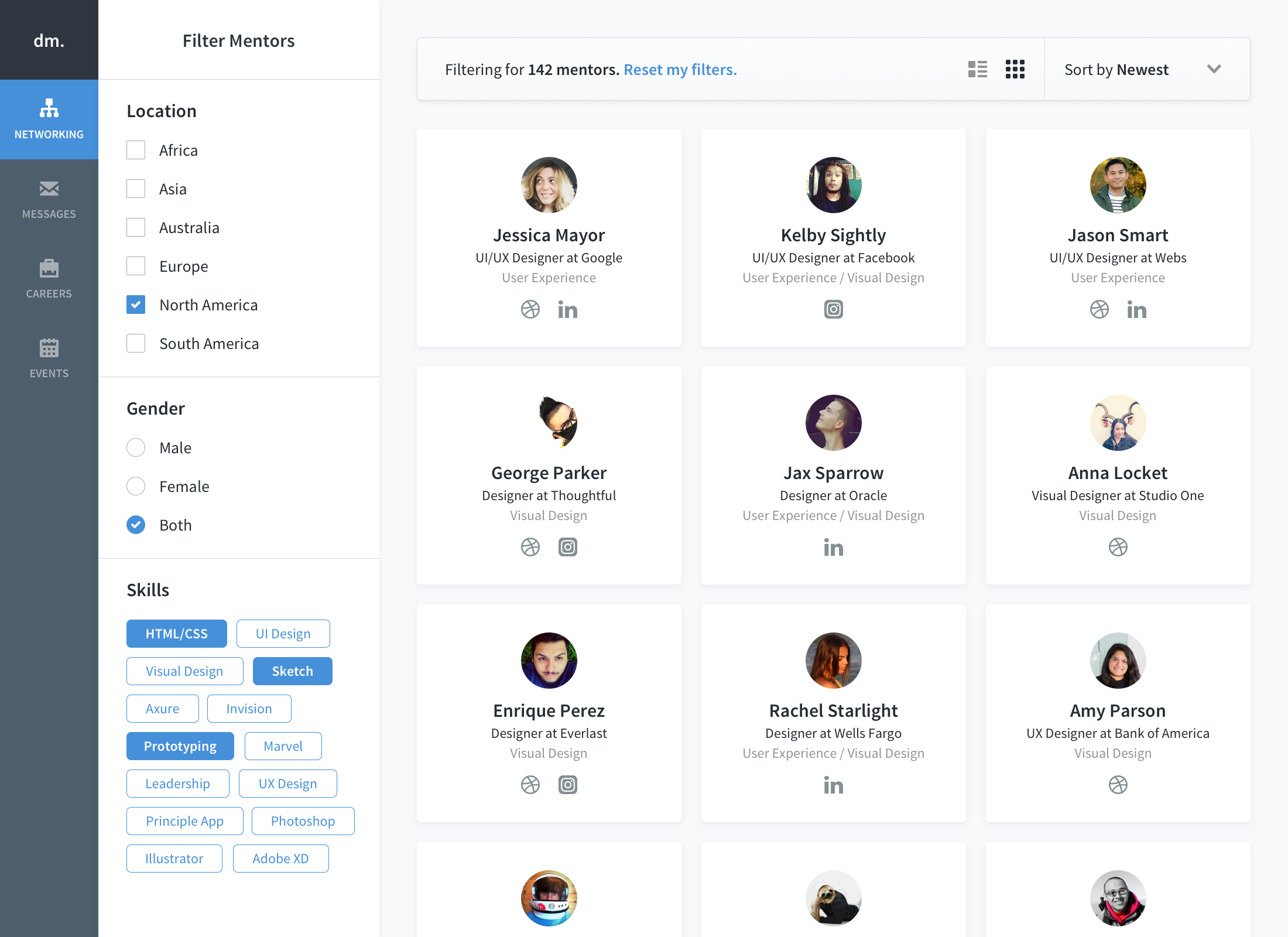The image is a screenshot of a user interface displaying various employees from different organizations, presumably mentors. On the left side, there is a filter section. At the top of this section, it says "Filter Mentors," and below that, the categories of filters are listed. The first category is "Location," offering options of Africa, Asia, Australia, Europe, North, and South America. The option for North America is selected. The next category is "Gender," with the option "Both" indicated, allowing for any gender to be included. The final category is "Skills," listing HTML, CSS, Sketch, and Prototyping. 

To the right, the results pane indicates the outcome of the applied filters, showing "Filtering for 142 mentors" at the top. The filtered list of mentors begins with Jessica Mayer, followed by Kelby Seidling, Jason Smart, George Parker, Jax Sparrow, Anna Lockett, Enrique Perez, Rachel Starlight, and Amy Parrison. Though there are three more mentors listed, their names are not visible, only their profiles can be partially seen. 

This detailed interface allows users to conveniently narrow down potential mentors based on specified filters, aiding in a targeted search for mentorship.